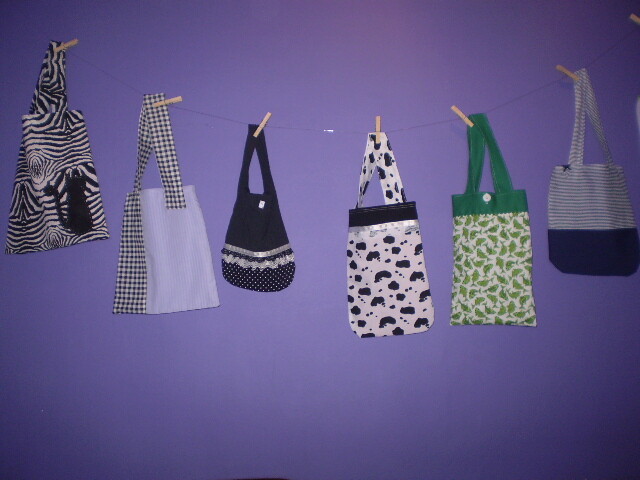This photograph shows six distinct cloth tote bags, carefully hung on a wire with wooden clothespins against a solid purple wall, captured with flash photography that highlights the center and fades out towards the edges. 

From left to right:
1. A black and white bag showcasing an almost zebra-like stripe pattern with a silhouetted black cat sitting in the bottom right corner, its ears and curled tail clearly visible.
2. A tote featuring a black and white checkered bottom half and a pale blue upper half, adding to its contrasting design.
3. The third bag is notably smaller and primarily black, with a lace ribbon encircling the middle. The bottom section is adorned with shimmery white beading details.
4. This rectangular bag has a white background with black blotches spread across it, resembling a Dalmatian pattern.
5. Predominantly green, this bag has congested leaf patterns on a white background. Its handle and top trim are solid green, completing its natural theme.
6. The final bag on the far right features thin horizontal blue stripes on a white background, with a navy blue bottom half, giving it a somewhat nautical appearance.

All the tote bags hang neatly from the wire, creating a visually appealing arrangement against the vibrant purple backdrop.